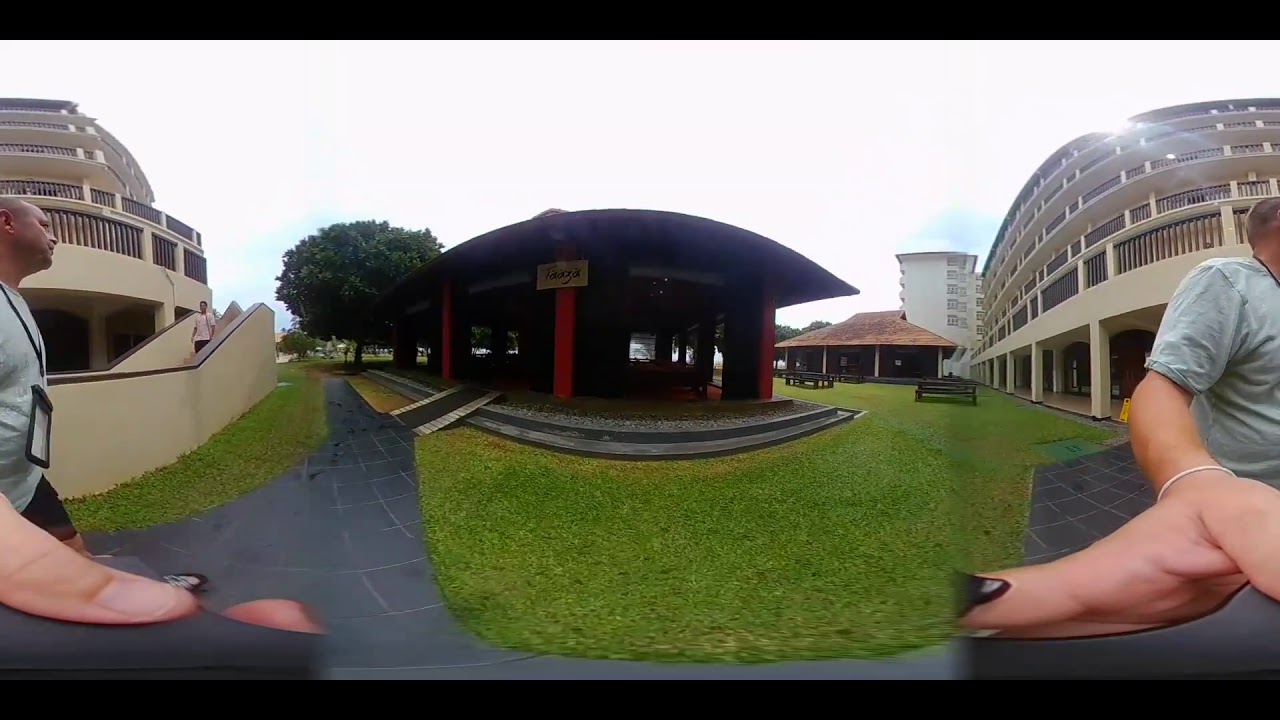In the fisheye perspective outdoor image, a red domed building with prominent red piers stands in the middle of a park-like courtyard. This central building, marked with "FAZA" written on it, is surrounded by a grassy area and a gray platform. To the left, there is a multi-storied white building with a ramp, and a man in a gray shirt with a tag is descending the steps. On the right side, another multi-storied off-white cream building features windows and benches scattered nearby, resembling an old McDonald's with a brown roof in the background. Additional details include a vertical white building without windows and a tree behind the central red building. The image curiously captures the same man, wearing a green short-sleeved t-shirt and an ID badge, partially visible on both sides as he walks through the scene, seemingly a result of the curved lens effect.